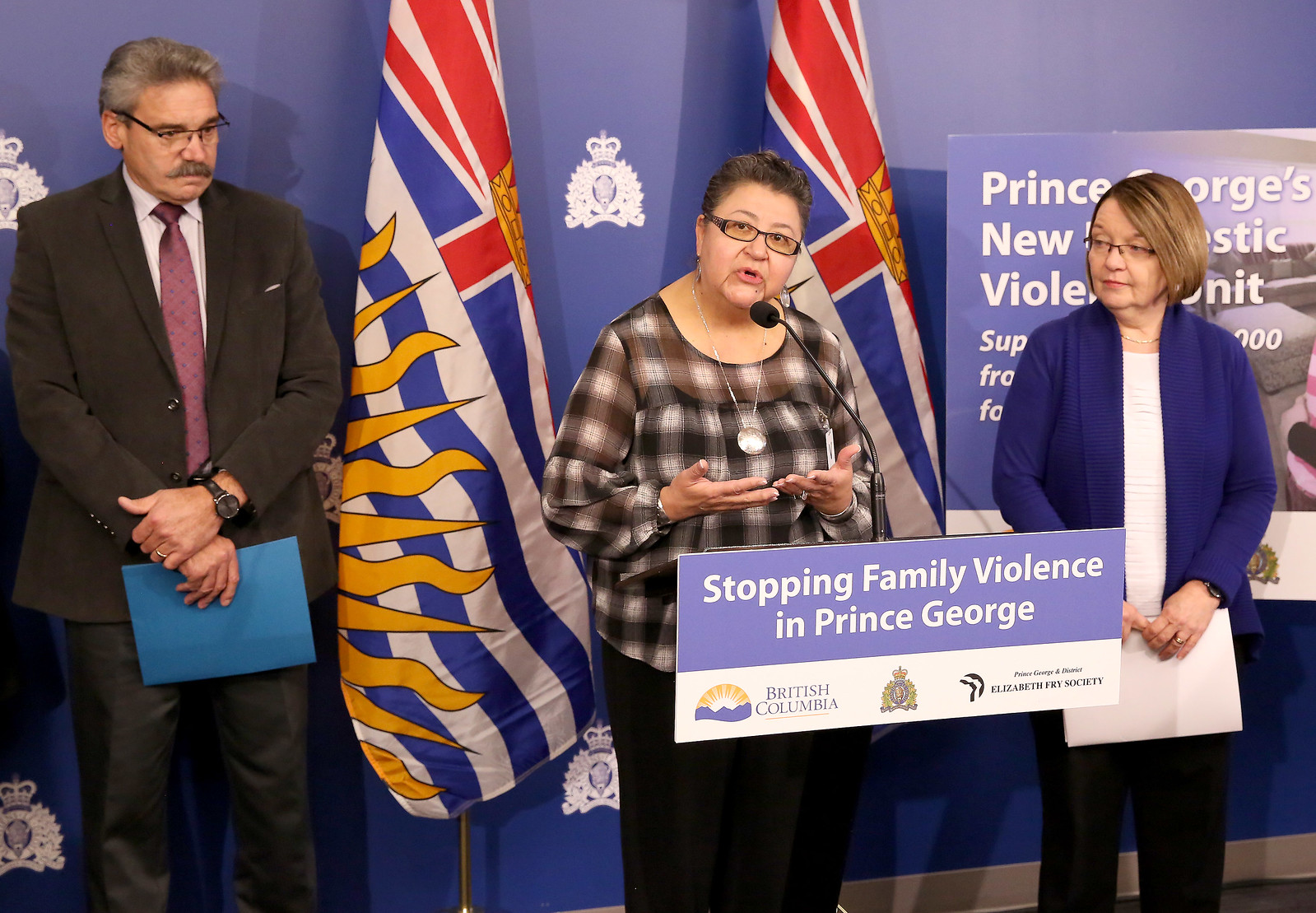The image captures an indoor scene set against a backdrop of repeated emblems on a blue wall. At the center of the photo, a short-haired woman stands behind a podium, delivering a speech. The podium features a rectangular banner with a purple and white background reading "Stopping Family Violence in Prince George, British Columbia." The woman speaker is gesturing with her hands and is dressed in a patterned long-sleeve shirt in white and gray hues, along with dark pants. She is flanked by two individuals; to her right is a woman in a bright blue jacket with a white shirt underneath and black pants, holding a piece of paper and looking towards the speaker. To her left stands a man in a black suit with a red tie and eyeglasses, also focusing on the speaker. Both women and the man are wearing eyeglasses. Two flags with colors including white, blue, yellow, and red are positioned behind the speaker, further framing the scene which appears to be part of a formal event or conference dedicated to addressing family violence.